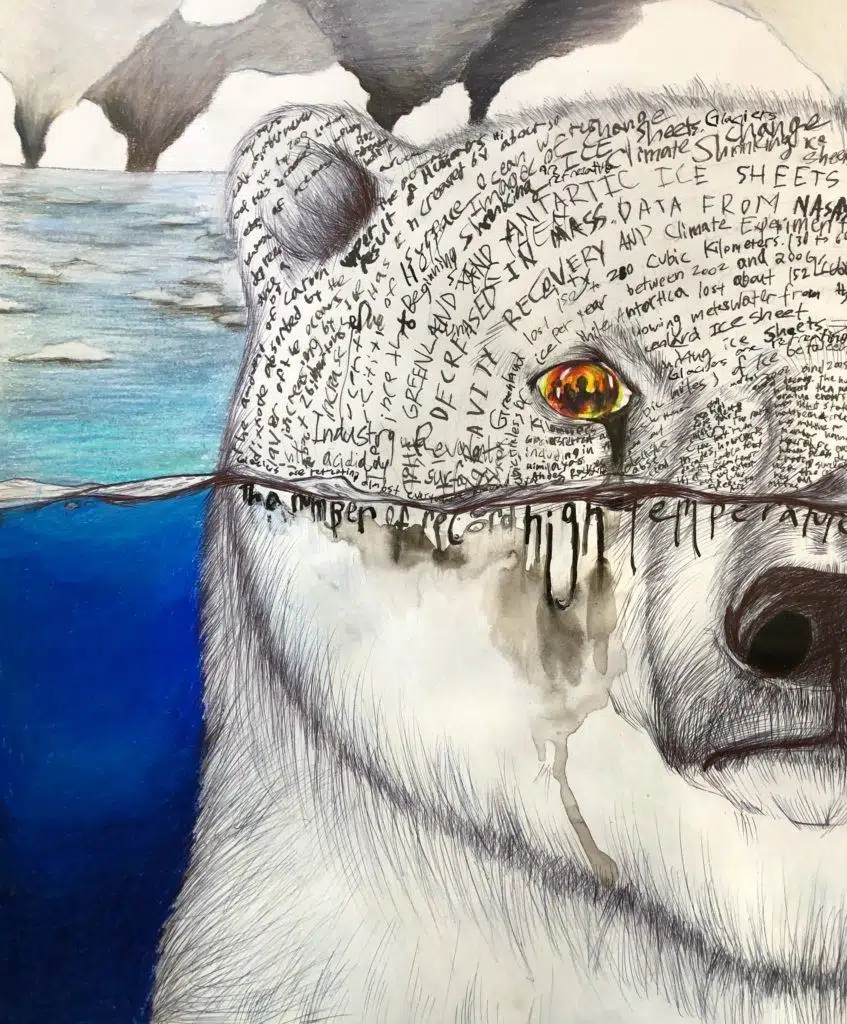This is a watercolor painting of a polar bear's face and neck, blending elements of abstraction and realism. The white and slightly gray bear is depicted with a large black nose and a single gold-yellow eye, which contains the silhouettes of human heads. The polar bear appears to be crying, and the smudged tears blend into the painting. The bear is partially submerged in a deep blue ocean, with its nose below the waterline and its eye above it, set against a subtle light blue sky. Above the bear’s nose and eyes are numerous writings, including text about Arctic ice sheets, climate change, and global warming, done in both handwriting and cursive. The background features black tornado-like shapes and ice crystals, enhancing the overall surreal and thought-provoking theme of the artwork.